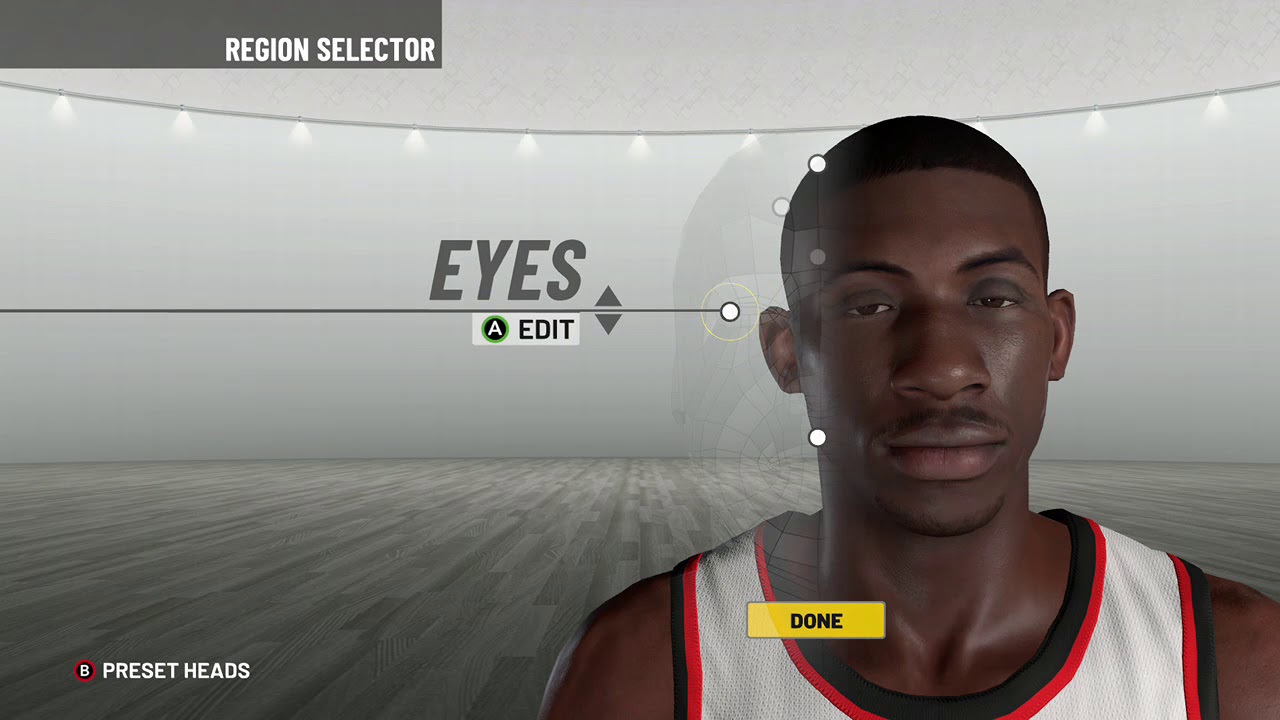In the game’s character generator interface, a unique, detailed design welcomes the player. The background is a neutral gray, setting a subdued tone, highlighted by a dynamic, slightly arched light beam that traverses from left to right, adorned with approximately 10 small luminescent bulbs hanging below it.

In the upper-left corner, a dark gray rectangle prominently displays "Region Selector" in clean, white text. Below this, a horizontal gray line extends from the left edge to the middle of the screen. Just above this line, the word “Eyes” is labeled in gray text, with an interactive circular A button and the word "Edit" directly below, drawing attention to a facial customization option.

Dominating the bottom right of the screen, the character preview showcases an African American male avatar. This character features brown skin, black hair, and expressive brown eyes. His facial attributes are detailed with a broad nose, full lips, small ears, a slight goatee on his chin, and a subtle mustache above his upper lip. He is dressed in a white jersey accented with red and black trim, displaying his broad shoulders.

In the bottom left corner, the option "Preset Heads" appears in white text, ready to assist with quick character updates. This interface combines essential customization options with a clean, engaging visual presentation.